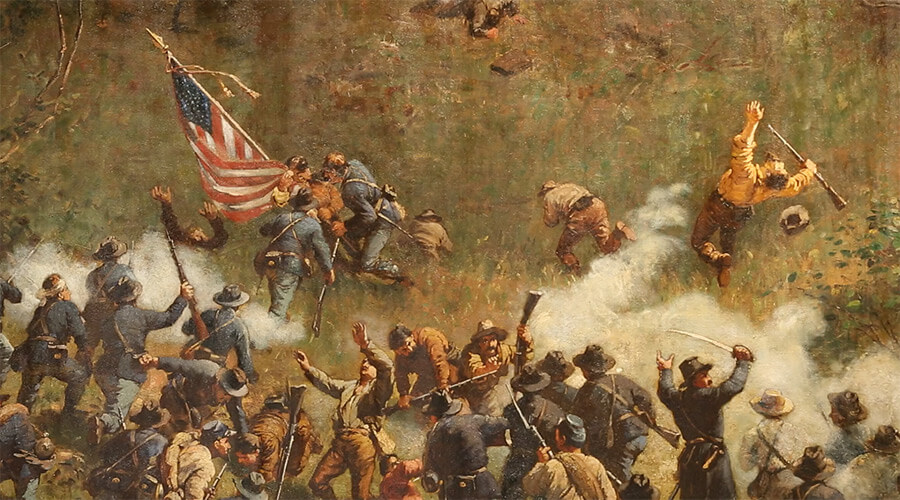This detailed image, likely a painting from the Civil War era, showcases a chaotic battlefield scene. The foreground is densely populated with soldiers, predominantly dressed in blue uniforms, indicative of Union troops, along with some in tan or gray uniforms, possibly representing Confederate forces. The soldiers are engaged in fierce combat, wielding muskets, swords, and rifles. One soldier can be seen holding a musket aloft in his right hand, while another falling backwards, dressed in an orange shirt and brown pants, clutches his rifle.

Central to the composition is a prominent American flag, held high by a soldier situated near the top left of the scene. This soldier appears to be amidst a surge of opposing forces. To his left, two soldiers in brown uniforms rush forward, adding to the tension of the battle.

Scattered throughout the bottom of the image are various skirmishes, with soldiers actively firing their weapons or engaging in melee combat. Amidst this disorder, several soldiers appear to have been struck, either falling or lying on the ground. Multiple clouds of smoke rise from these encounters, contributing to the atmosphere of chaos.

The backdrop of the painting is a mix of faded green and brown hues, suggesting a grassy terrain or village landscape, partly obscured by the smoke of battle. Overall, the painting vividly captures the tumult and intensity of a Civil War battle, with a focus on the crowded and frantic lower section teeming with combatants.